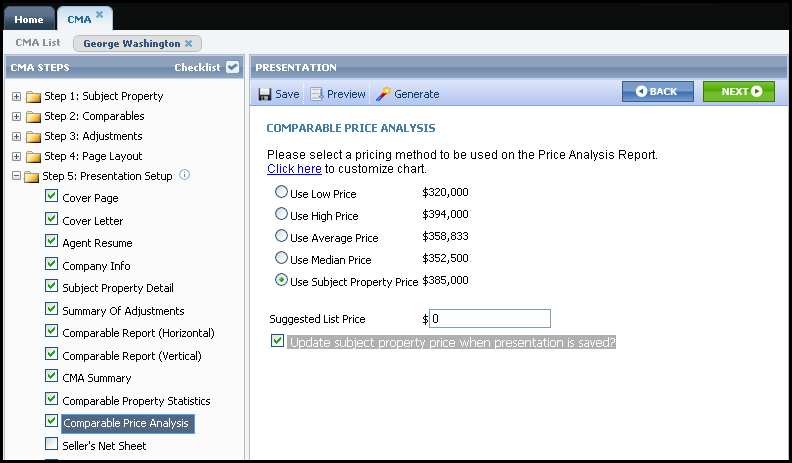A cropped screenshot of a company software interface shows two tabs at the top: "Home" and "CMA." The "CMA" tab, indicated in blue, is currently active. The primary section of the screenshot features a large, white rectangular box against a black background, with a black border around all four edges, significantly thicker at the top.

Below the tabs, the screen displays a "CMA List" with a text box containing "George Washington." To the left, there is a long rectangular panel titled "CMA Steps" on the upper left and "Checklist" on the upper right. This checklist includes a checkmark, indicating completion.

The "CMA Steps" section lists five steps, with Step Five expanded to reveal all its subcategories. The subcategory "Comparable Price Analysis" is selected. On the right side of the page, the section is open to this analysis, with instructions to "Please select a pricing method to be used on this price analysis report." The statement "Click here to customize chart" is hyperlinked.

Below this, there are clickable buttons arranged on the far left, followed by options to the right, and amounts listed on the far right. At the bottom of the screen, there is a blank text box labeled "Suggested List Price" for input, accompanied by a checked box that says "Update subject property price when presentation is saved."

This detailed structure of the software interface provides a comprehensive overview of the current module in use.